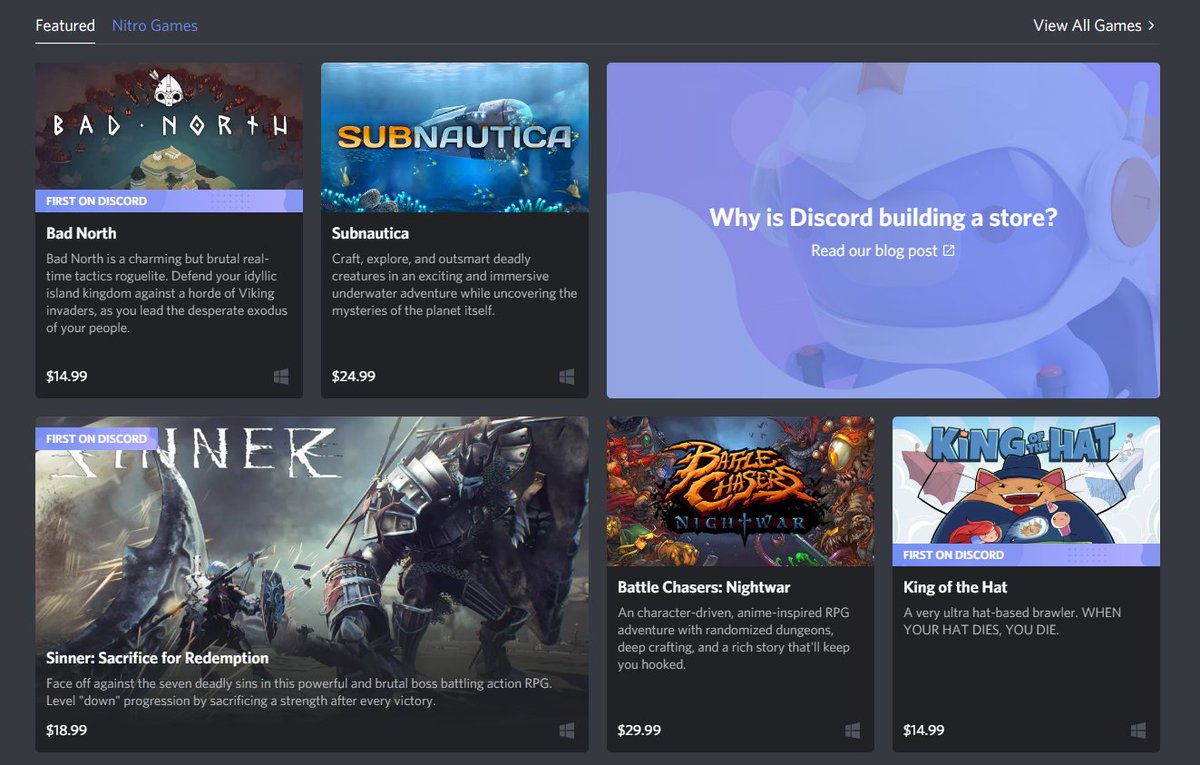The image showcases a dark-themed digital storefront, reminiscent of Steam, dedicated to video games. This platform appears to be part of Discord, identifiable by the prominent Discord logo and app interface integrated into the upper right corner. The storefront is displaying the 'Featured' tab, one of the two available tabs along with 'Nitro Games'. Several indie games are listed, including 'Bad North', 'Subnautica', 'Sinner', 'Battle Chasers', and 'King of the Hat', with 'Bad North' and 'King of the Hat' marked as "First on Discord" exclusives. 'Subnautica' is priced at $25. The platform specifically supports Windows, as indicated by the Windows icons next to each game listing. A 'View All Games' button is located at the top right corner of the interface. The presence of an announcement about a retirement blog post raises curiosity about Discord's venture into game retailing.